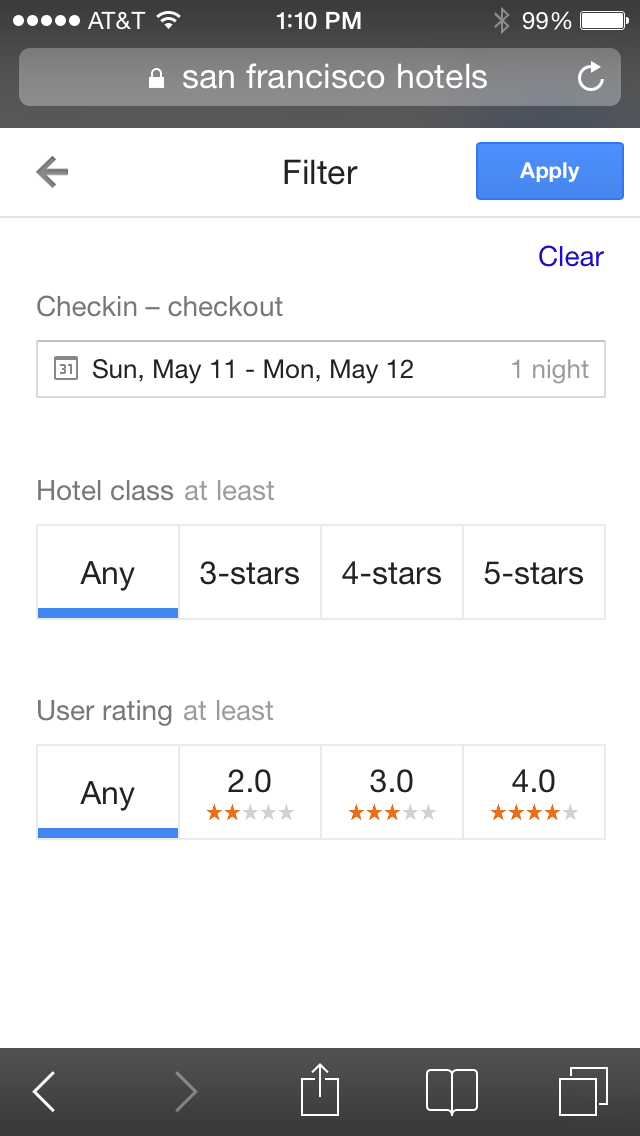This is a screenshot taken on an AT&T mobile phone that shows a full signal and a fully charged battery. The time displayed is 1:10 p.m. The screen is currently displaying a search for hotels in San Francisco. Below the search result header, there is a navigational arrow pointing to the left and a button labeled "Filter." Adjacent to this button is a blue button that says "Apply."

The search criteria include check-in on Sunday, May 11th, and check-out on Monday, May 12th, making it a one-night stay. The filter settings show that the hotel class is set to include any rating from three to five stars, with the "Any" option currently selected. User ratings are also set to include any rating from two to four stars, with "Any" selected as well.

At the bottom of the screen, there are several icons: a left-pointing arrow, a right-pointing arrow, a page icon with an upward arrow, a split-screen view, and an icon depicting pages slightly overlapping each other. The user chose the "Any" options for both hotel class and user rating, which might seem surprising to some.